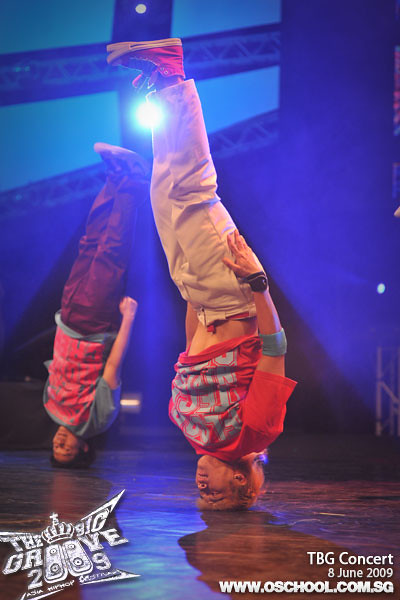In the narrow, vertical, and somewhat blurry image, two men are performing a headstand on a stage, their arms extended straight alongside their bodies. Both individuals are positioned upside down with their feet pointed upwards, demonstrating a level of difficulty in their stance. The stage has a wooden floor and a blue backdrop, illuminated by a spotlight shining down the middle, highlighting their precise posture. The man in the background wears a blue t-shirt with large pink text, black pants, and tennis shoes. He has short black hair. The man in the foreground sports short blonde hair, a red t-shirt with large blue text, khaki pants, and red Converse shoes which reveal a bit of his midsection. At the bottom of the image, there are two pieces of text; the lower left corner reads "Magic Groove 2009" while the lower right corner presents "TBG Concert, 8 June 2009, www.oschool.com.sg" aligned in white print. This scene appears to be part of a dance performance, possibly a stunt showing strength and balance, occurring during a concert event.